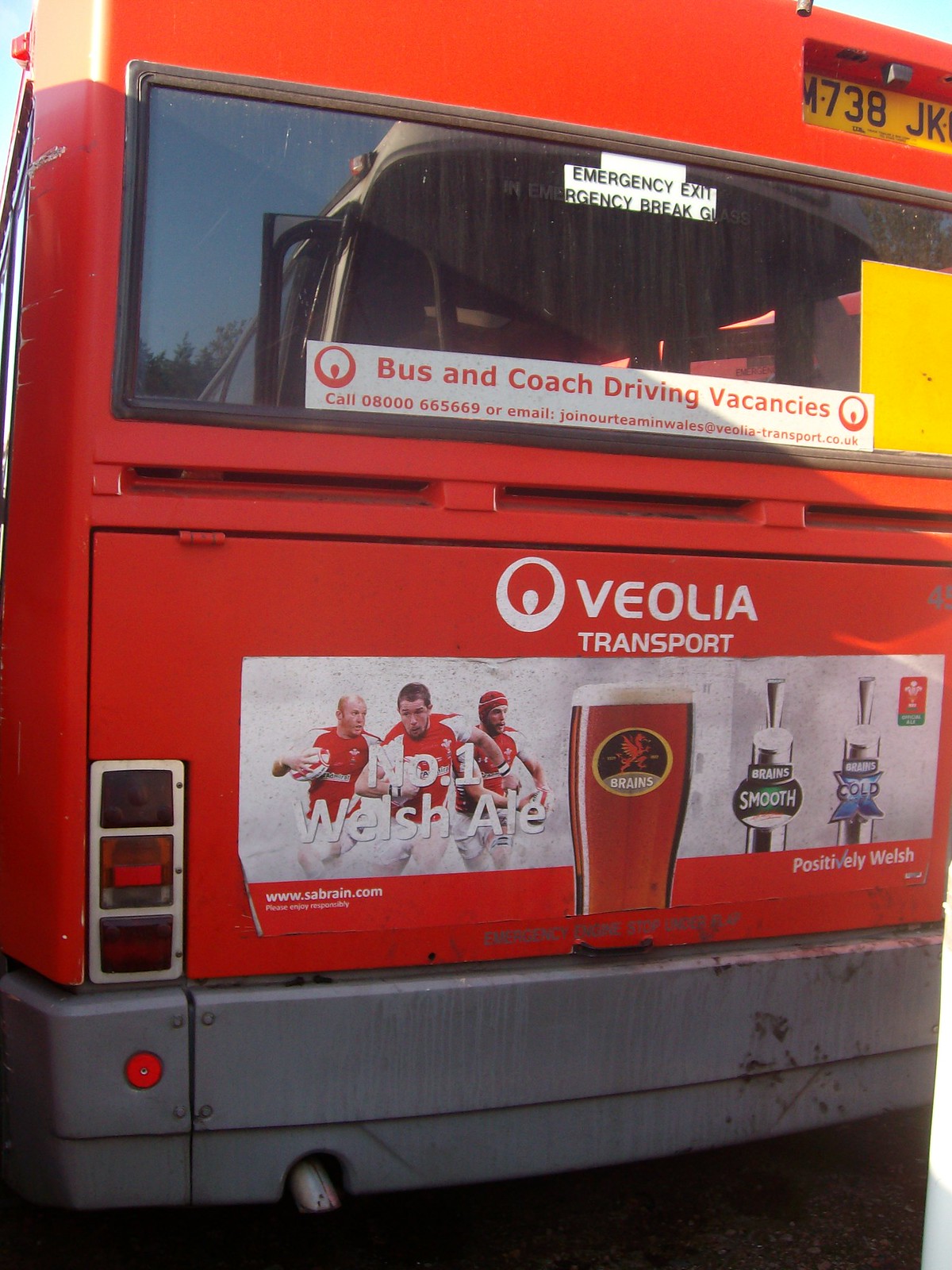The image captures a detailed close-up of the back of a red city bus. Dominating the top section is a yellow license plate which reads “N738JK,” just below the red upper part of the bus. Adjacent to the license plate, to the left, is a backlight. The most prominent feature is a large black window with several stickers. At the top of the window is a notification that says, “Emergency Exit – Emergency Break Glass.” Below this, on a white background with red text, there is an advertisement reading, “Bus and Coach Driving Vacancies. Call 0800 066 5669 or email join our team in Wales at veolia-transport-co-uk.” 

Beneath this ad, the logo for Veolia Transport is displayed, a thick white circle with a dot in the center, accompanied by the text “Veolia Transport.” Further down, dominating the middle section, is an ad for a beer, depicting three men in white and red shirts playing an unspecified sport alongside text stating, “#1 Welsh Ale.” Centered in this ad is an image of a golden-colored ale with the brand name “Brains.” To the right of the beer image are two beer spouts with the phrase “Positively Welsh.” The lower portion of the bus includes a grey bumper, and a little pipe can be seen protruding from below the bus.